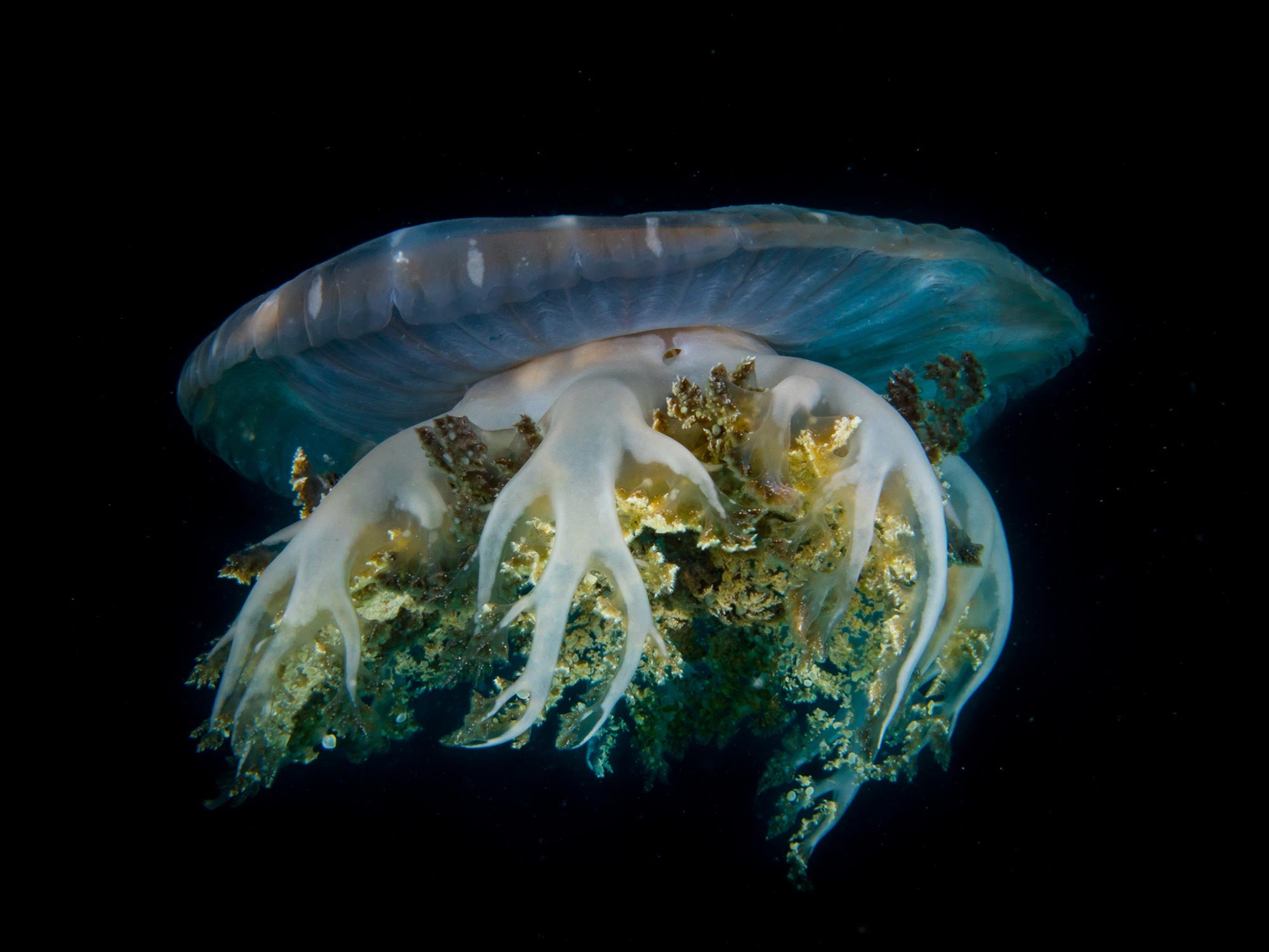This image features a close-up view of what appears to be a Portuguese man o' war or possibly a jellyfish, set against a solid black background. The creature is visually striking, with a transparent, light blue "jelly" part forming the top or main body. This section exhibits accents of orange and faint traces of yellow and green, giving it an ethereal quality. Below the blue body, long, white tentacles extend downward, intricately detailed with structures that resemble flower petals or algae. These structures transition from bluish hues at the bottom to yellow and greenish shades higher up. There is no text in the image, and the overall appearance is so vivid and detailed that it almost looks digitalized or altered, despite being a real photograph. The background's dark tone enhances the creature's vibrant colors and intricate features, making it the focal point of this mesmerizing and beautifully captured photo.